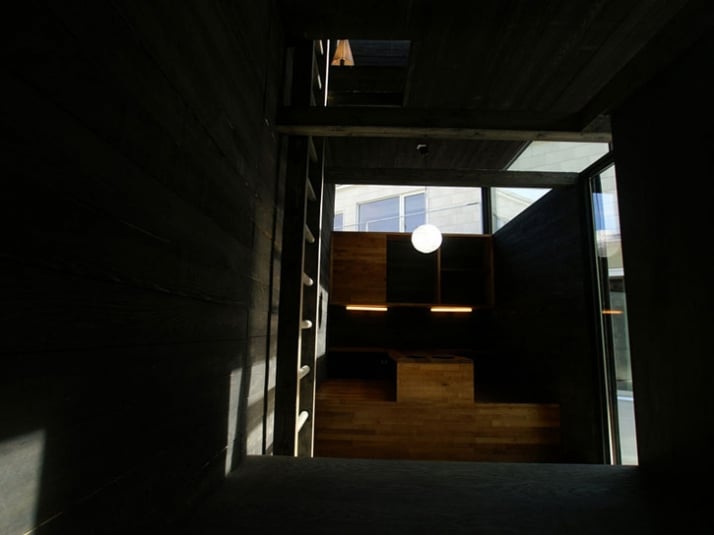The image depicts an interior scene viewed through a window, presumably taken with a camera flash as evidenced by the bright hot spot in the center. The exterior appears illuminated, suggesting daylight, while the space inside is dimly lit and appears small and intimate. On the left side, a wooden staircase ascends, and just past it, a wooden ladder with cylindrical rungs is mounted on the wall. The flooring inside is composed of wood planks, extending towards the far end of the room where two small, long, cylindrical lights are mounted under a set of wooden shelves.

In the center of the ceiling, a lighting fixture dangles above what appears to be a small, low table, possibly designed for sitting cross-legged around it. This table seems to be an integral part of the floor, requiring a step up to reach it. The far end of the space features windows, located high on the wall, allowing a glimpse of a beige brick building outside, which could be either a residential or commercial structure with large windows.

Overall, the image captures a cozy space with various wooden elements and minimal light, contrasted against the brighter, indistinct exterior visible beyond the window.